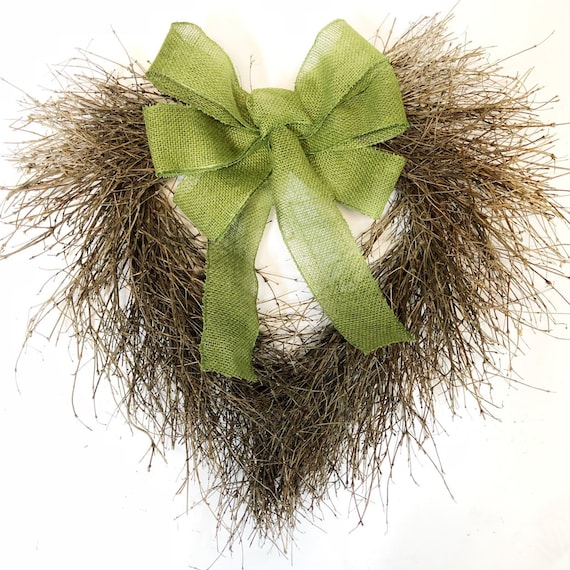The image features a heart-shaped wreath crafted from thin, brown, dried branches or fiber, giving it a natural and rustic appearance. It is meticulously centered against a plain white background, which enhances its contrast and focus. Adorning the wreath is a large, decorative bow in a light green, almost sage or lime hue. The bow is intricately designed with six loops—three on each side—and two trailing ribbons that elegantly extend downward towards the midpoint of the heart. The central positioning of the bow between the two arches of the heart adds a delicate touch to the overall composition, creating a visually appealing craft item devoid of any text, people, or additional colors.